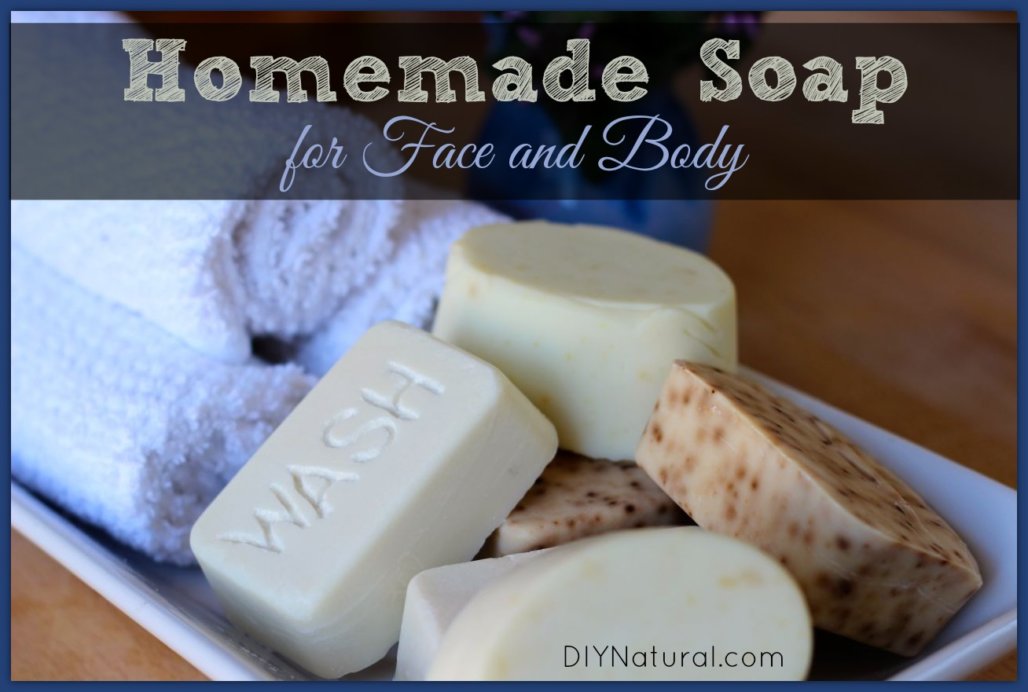In this image, we see a detailed arrangement of artisanal soaps and towels set on a white ceramic tray, which is placed on a wooden platform. The display includes six bar soaps: four milky white and two brown, with one of the brown soaps featuring black and brown specks. One soap has the word "wash" imprinted on it and is rectangular with rounded edges. The soaps appear handmade and natural, designed for face and body care. 

Beside the soaps, there are three neatly rolled white towels, showing a slight bluish tint. The entire composition is framed with a thin blue border, enhancing the calm and clean aesthetic of the scene. 

At the top of the image, a semi-transparent black banner with chalkboard-like text declares "Homemade Soap for Face and Body," with the latter part in a light blue cursive script. At the very bottom, the URL "DIYNatural.com" is presented in a thin black font, providing a source for these delightful creations. There is also a blurry blue item in the background, adding a subtle depth to the scene. The overall image is designed with a blue-tinted frame that complements the serenity and natural appeal of the display.